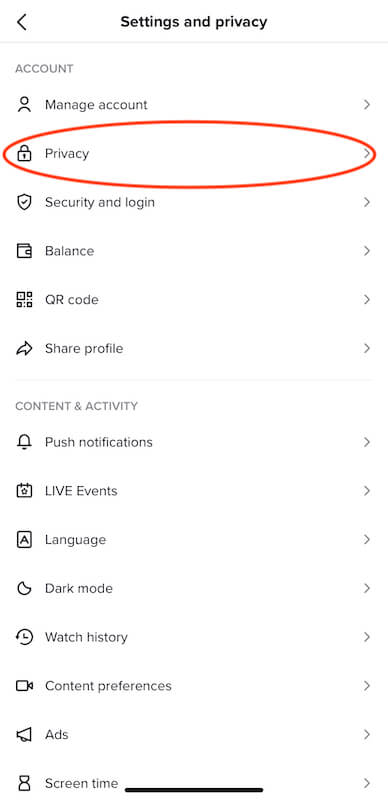This image is a detailed screenshot of a mobile phone's "Settings and Privacy" menu, displayed against a white background. At the very top center is the heading "Settings and Privacy" in black letters, with a small arrow on the left side. Below this heading is a comprehensive list of settings categories and options.

The first category is labeled "Account". Under this, various options are listed:
1. Manage Account
2. Privacy (which is circled in red)
3. Security and Login
4. Balance
5. QR Code
6. Share Profile

A narrow white space separates the "Account" section from the next category, "Content and Activity". The options under this category include:
1. Push Notifications
2. Live Events
3. Language
4. Dark Mode
5. Watch History
6. Content Preferences
7. Ads
8. Screen Time

Each option is accompanied by a small icon on its left and an arrow pointing to the right on its far right side, providing a visual indicator for further navigation. At the very bottom of the screenshot, a black line demarcates the end of the visible settings menu.